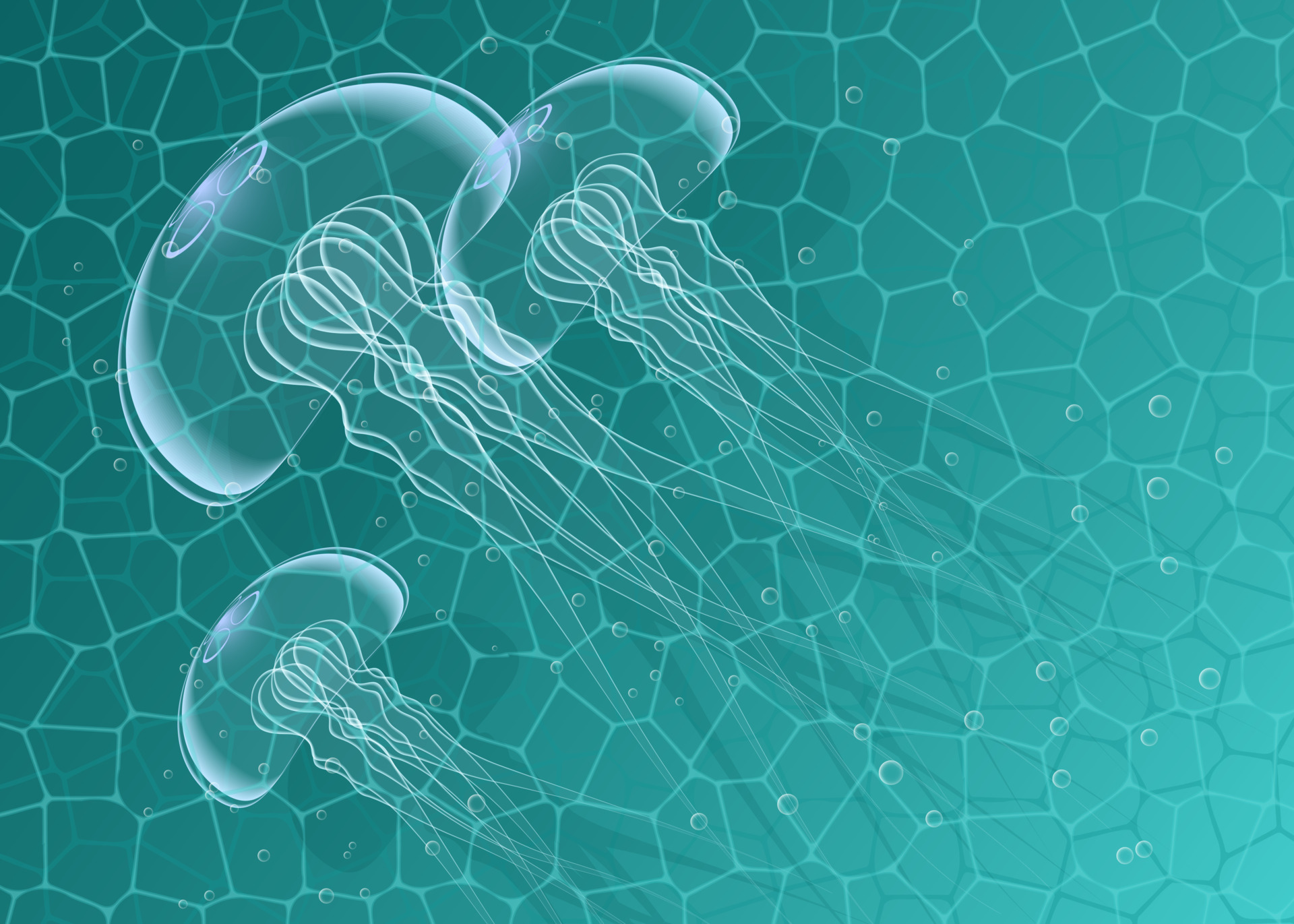The image is a detailed 3D rendering of three semi-transparent jellyfish swimming in a marine setting. The rectangular frame features a dark blue background with a geometric grid made up of light blue hexagonal and trapezoidal shapes. Each jellyfish, with its large, globular, half-circle-shaped body, is orientated towards the top left corner, creating a dynamic sense of movement across the image. The semi-transparent tentacles, which are both within and extending beyond the jellyfish bodies, give a delicate, ethereal feel. The background includes subtle shadows of the jellyfish, enhancing the depth, along with multiple white transparent circles representing bubbles, adding to the underwater atmosphere. The intricate design captures the essence of marine life, with an emphasis on the transparent, wiry, and flowing nature of the jellyfish's tentacles moving gracefully within the aquatic environment.